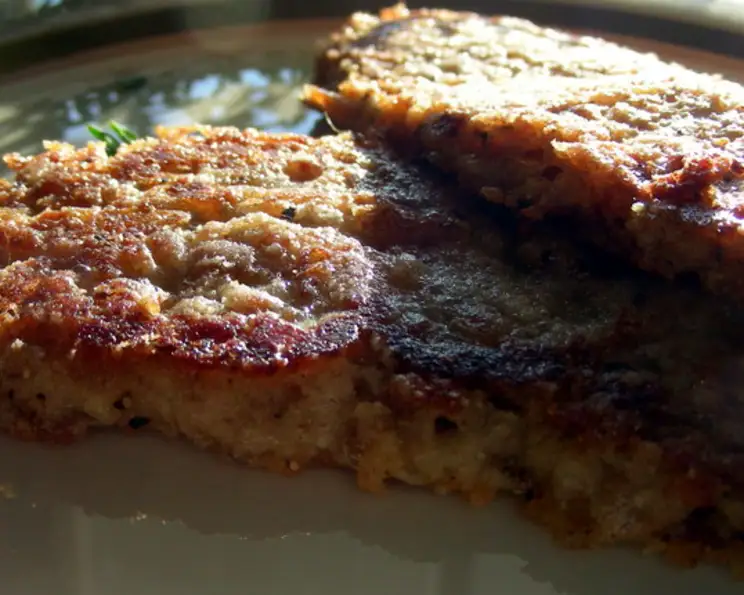This close-up image displays a dish of what appears to be breaded and pan-seared cutlets, arranged attractively on a white plate with a black and white rim. The cutlets have an enticing sear, with a brownish-red and slightly darker golden-brown crust, suggesting a well-cooked surface. The dish features two main cutlets, positioned one atop the other in an opposite direction. Near the back left of the lower cutlet, two green petals, possibly a garnish, peek out, adding a touch of color. The center of the dish exhibits an orange hue transitioning to a red edge, creating a visually appealing contrast against the predominantly golden-yellow crust. The lighting highlights the left side of the plate, casting a shadow on most of the cutlets, enhancing the textured details of the dish.